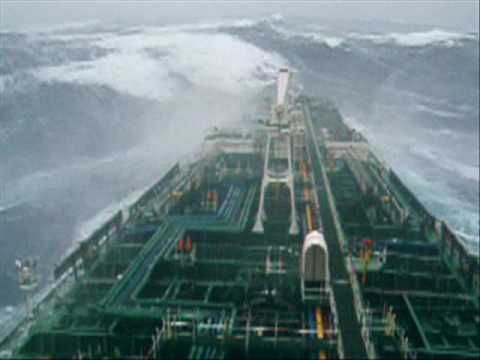The image shows a large tanker ship navigating through stormy seas. The vessel's deck is lined with extensive pipework, including four pipes running along the left side and several more spanning the width of the ship. The seas are incredibly rough, with waves reaching heights of 15 to 20 feet, breaking over the bow, and splashing against the ship's sides. The entire scene is captured from a crow's nest or recording camera, lending a grainy quality to the image. The dark gray skyline and heavy rain contribute to the ominous atmosphere, emphasizing the harsh conditions. Whitecaps are visible across the choppy sea, and fortunately, the deck appears to be deserted, ensuring no crew members are exposed to the treacherous environment.